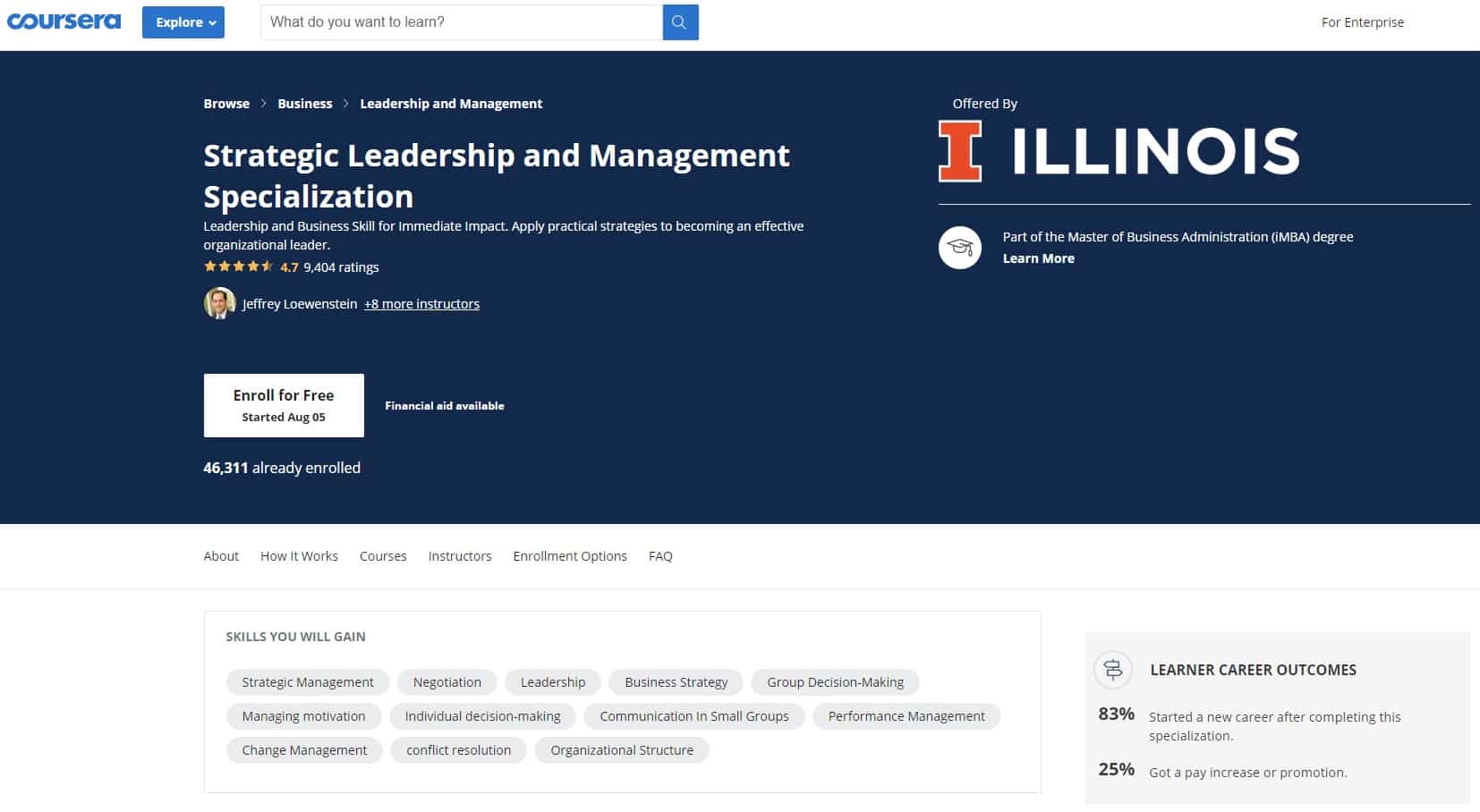**Screenshot of a College Website: Coursera Partnership with University of Illinois**

The image is a screenshot of an educational website, specifically from Coursera. In the upper left corner, the Coursera logo is prominently displayed. Centralized but slightly left-leaning on the page, the text reads "Strategic Leadership and Management Specialization." Below this title, there's a brief, slightly blurry description mentioning the acquisition of skills for immediate impact and the application of practical strategies to become an effective, organized leader.

On the right side of the page, it states that the specialization is offered by the University of Illinois. Just beneath that, it is noted that this course is part of the Master of Business Administration (MBA) degree. At the bottom, a white button with the text "Learn More" invites visitors to explore further details.